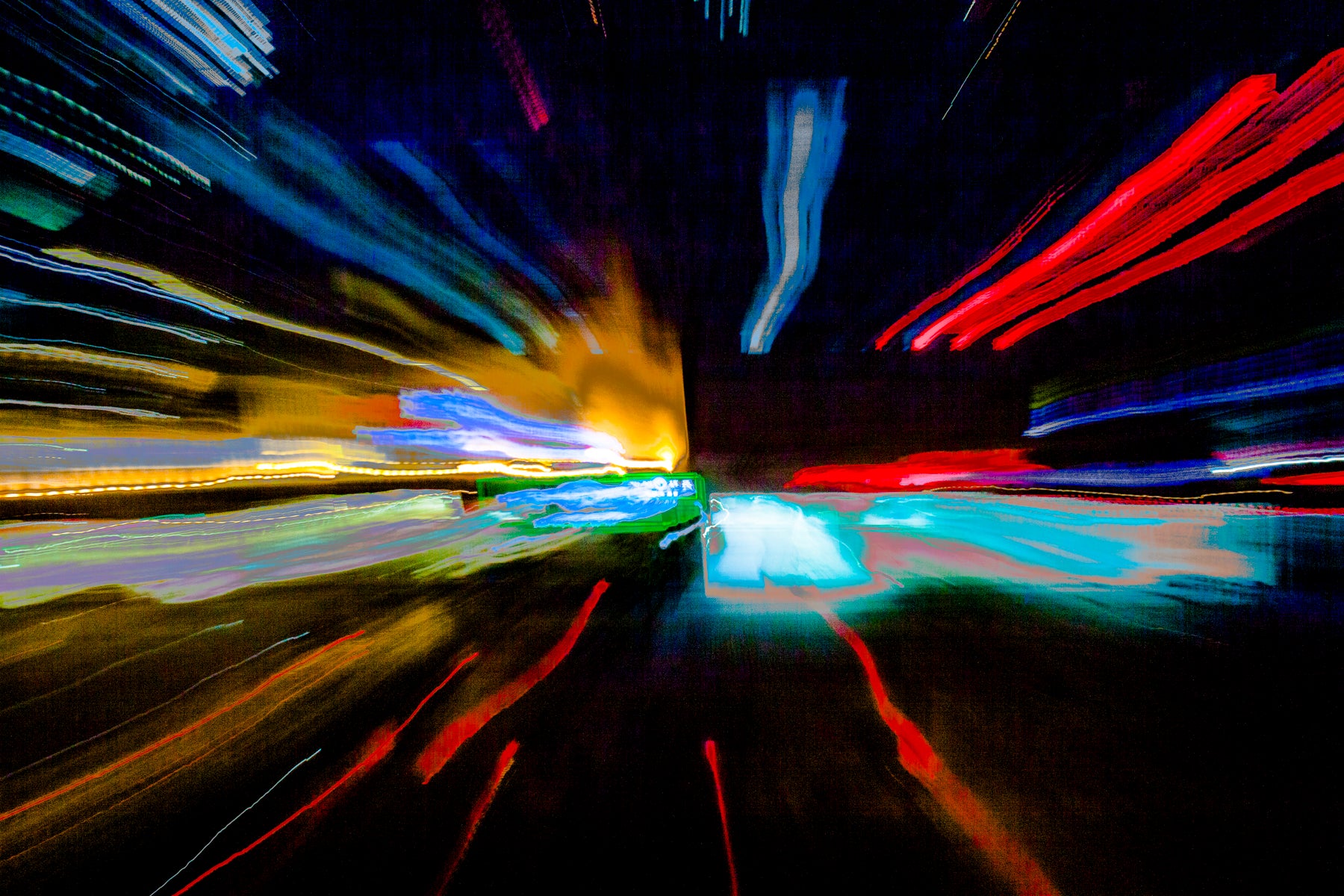This vibrant abstract painting features a stark black background that sets off a dynamic explosion of colorful rays. From the center of the image, there are streaks of bright colors such as red, blue, yellow, green, and teal radiating outward, creating a sensation reminiscent of blurred city lights seen from a speeding vehicle. The middle of the image is particularly illuminated with a blend of blue and green hues, giving way to red rays that extend towards the top right, bottom, and bottom left corners. Yellow and light blue streaks stretch from the center towards the left-hand side and top left. The painting is divided into distinct color quadrants, with each hue seeming to claim its territory while also blending into the next, adding to the painting's dynamic and fluid motion. This complex interplay of colors and movement captures the essence of high-speed visual experiences, rendering an energetic and mesmerizing abstract composition.